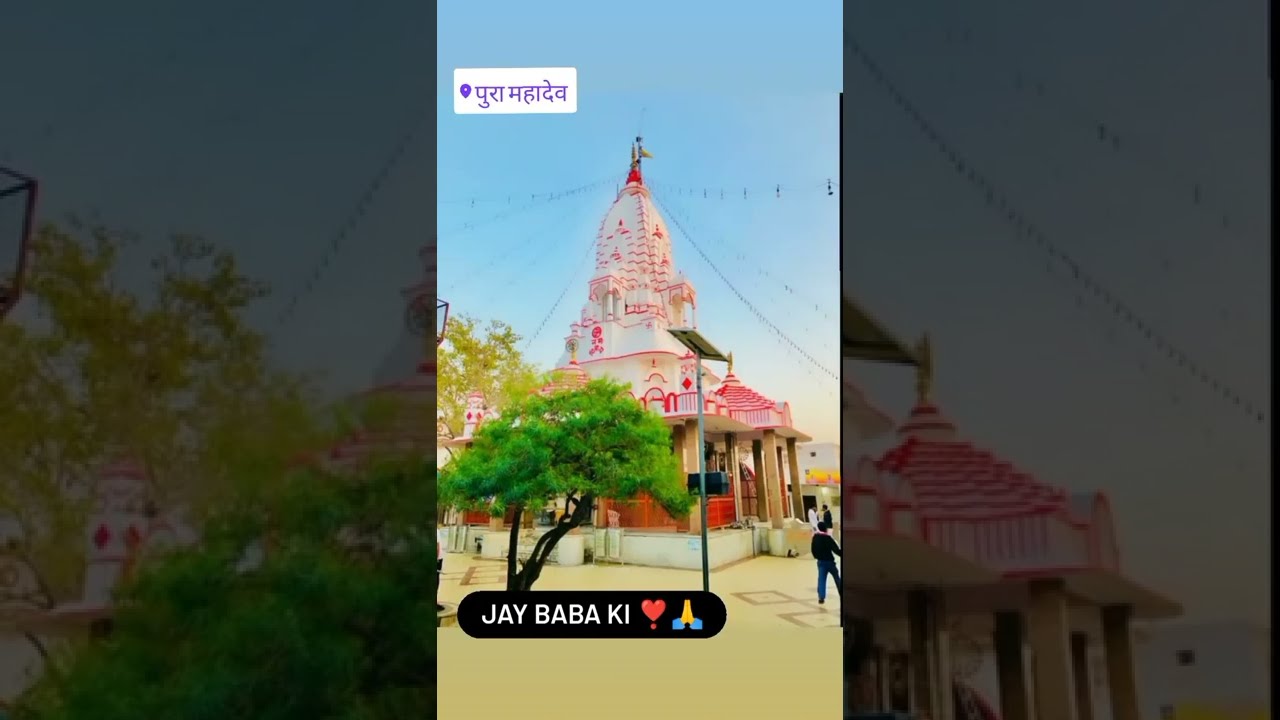The image captures a tall, ornate building that resembles a Hindu temple, predominantly white with intricate pink accents and details. The structure rises to a point where a gray statue, supported by various cables, is perched at the very top. The building is adorned with pillars and columns, and it has a white base trim. In front of the temple, partly obscuring its base, stands a small, green tree with rounded leaves and dark branches. The image is divided into three sections; the left and right sides are heavily tinted and zoom in on specific details: the right side focuses on the roof with visible columns and cables, while the left side highlights the tree and part of the building behind it. Above the temple, there is a white box in the upper left sky containing purple lettering in a foreign language, possibly a geolocation marker in Marathi. At the bottom of the photo, a black box reads "J-A-Y-B-A-B-A-K-I" followed by a red heart and clasped hands emoji. The scene is bustling with people walking around, indicating it was taken during the day.